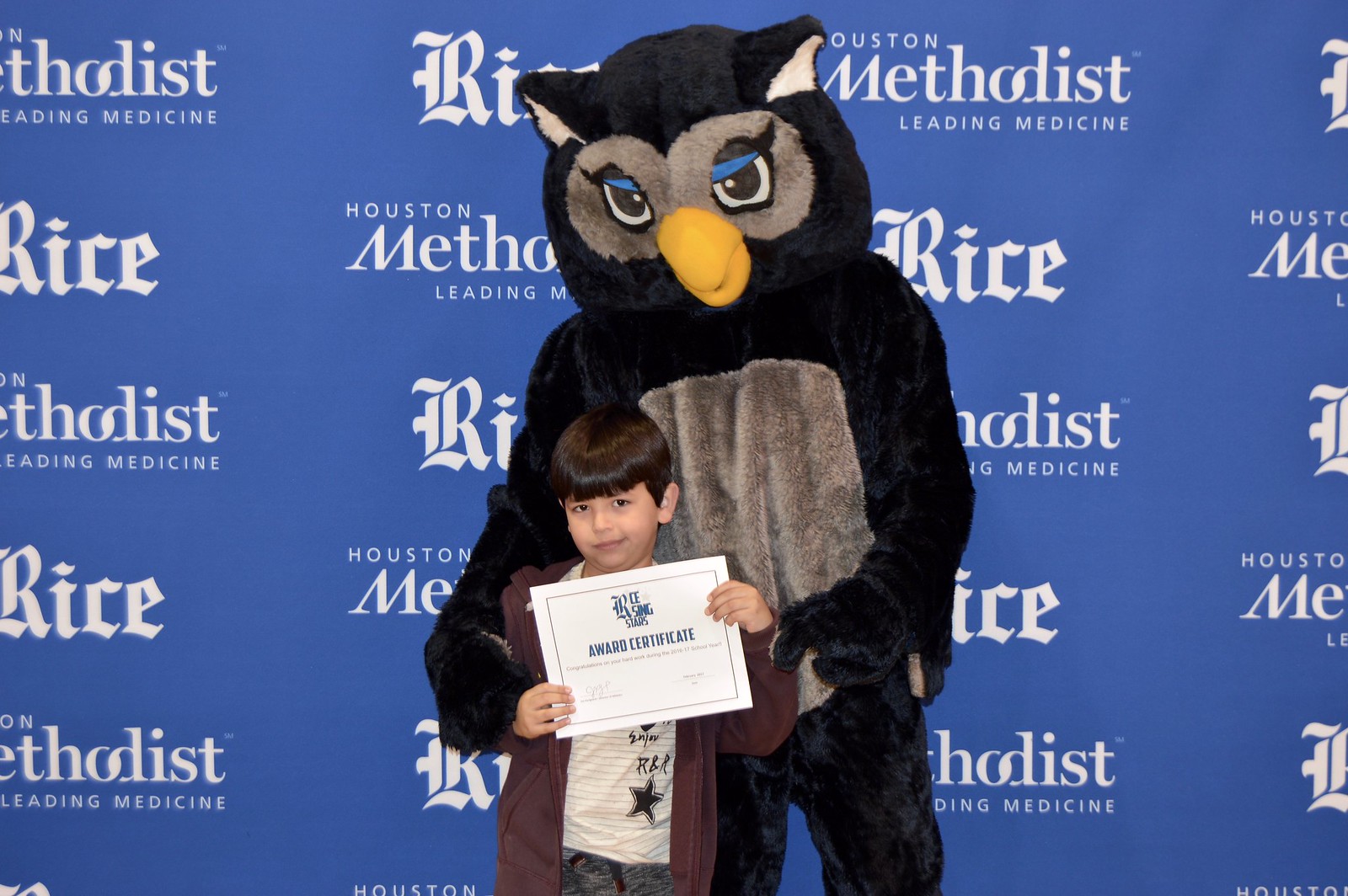In this horizontal photograph, a young boy stands proudly in front of a blue background adorned with repeated white text saying "Houston Methodist Leading Medicine" and "Rice." He holds an award certificate from Rice University in his hands, which are positioned slightly unevenly on either side of the paper. The boy, who appears to be around seven years old, has brown hair and is dressed in a burgundy or brownish jacket over a white t-shirt that features black stripes and the letters "R&R" with a star at the bottom. Standing behind him and enveloping him in a friendly gesture is a person dressed in a detailed owl costume. The costume is predominantly black with gray accents on the chest and around the eyes, a yellow beak, and white ears. The owl’s eyes are intricate, with blue and white detailing and black pupils, capturing the festive spirit of the event at Rice University in Houston, Texas.